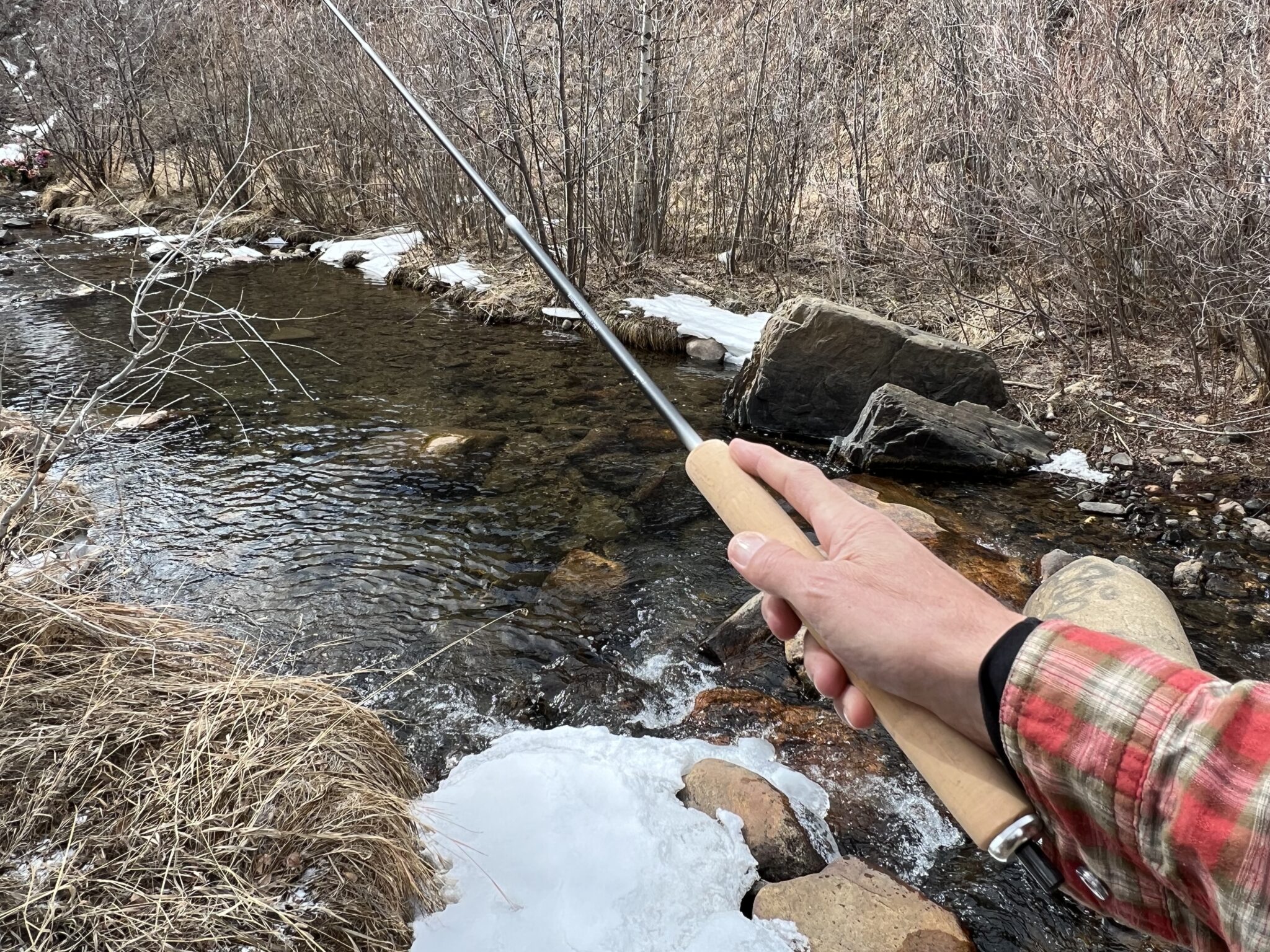In this outdoor winter photograph, a person is captured fishing in a clear, fast-moving stream winding through a dense, leafless forest. The image, taken from a point-of-view angle, shows a human hand emerging from the lower right, gripping a simple fishing rod with a tan, wooden handle and a black graphite pole structure. The arm, dressed in a long-sleeved black shirt and a red plaid flannel, extends the rod over the stream, flanked by thin, short deciduous trees and remnants of frost and ice. The person’s leg, clad in camouflage pants, adds to the scene’s rugged nature. The ground near the stream is covered in dead grass, and large stones peek from both beneath and above the water's surface, while patches of snow and ice dot the wintry environment.